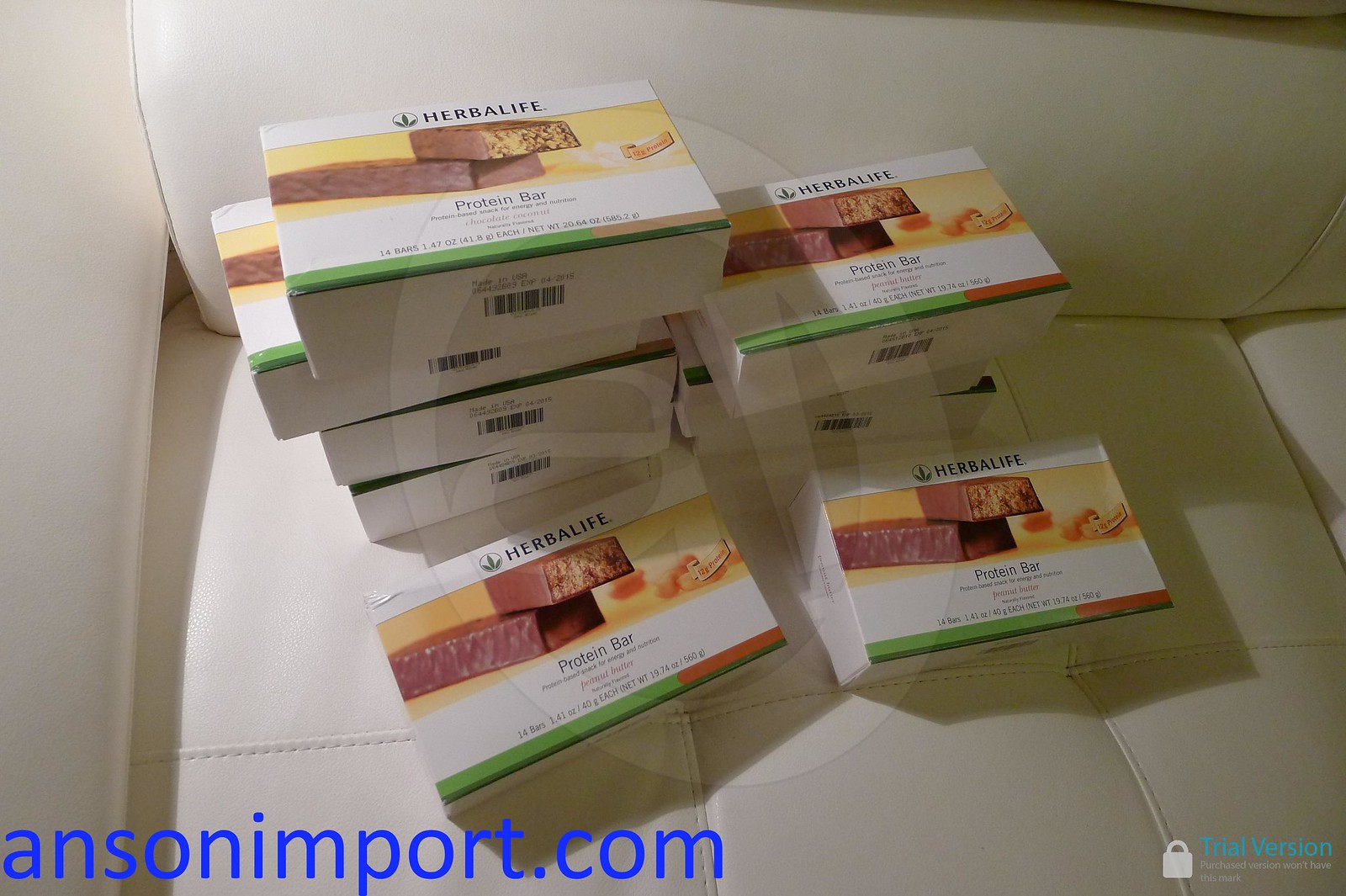The image features eight neatly stacked boxes of Herbalife protein bars arranged on a white leather couch. The couch has multiple top panels sewn together for each cushion and a single-piece cushion on the back. The boxes are predominantly white with images of chocolate-covered protein bars on their fronts and the Herbalife logo, which consists of a three-leafed emblem inside a circle next to the words "Herbalife." There are two stacks of boxes at the back, one stack with four boxes on the left and another with three on the right, with two additional boxes lying flat in front. On the bottom left of the image, the text "ANAONIMPORT.COM" is written in blue, though part of the URL appears incomplete. The bottom right corner features a watermark of a white lock icon with the text "TRIAL VERSION" also in blue. The boxes cast shadows on the couch, indicating some lighting from the top left. Additionally, each box has a visible barcode.